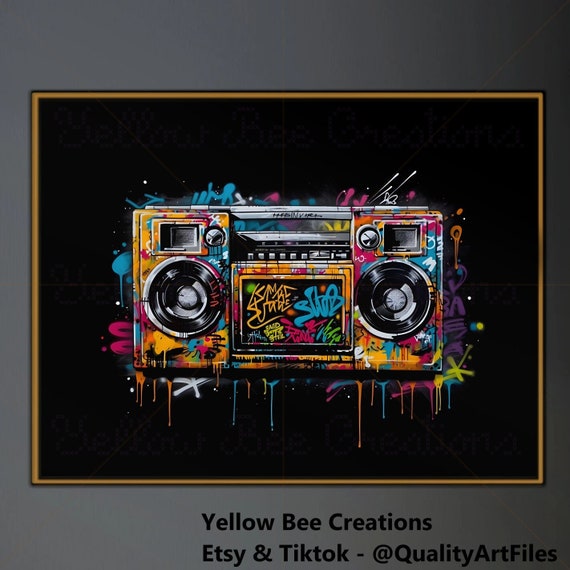This image is a vibrant, stylized cartoon drawing of an old-school boombox adorned with psychedelic graffiti. The boombox features a cassette player with push buttons in the middle and two circular black speakers on either side. Vivid colors—pinks, blues, oranges, greens, yellows, and reds—splash across the boombox, creating a dripping effect that adds to its dynamic appearance. Graffiti tags, though hard to read, add an edgy, street-art feel. The image is set within a thin gold frame, against a gradient background that transitions from lighter gray on the left to darker gray on the right. At the bottom, black text reads "Yellow Bee Creations," followed by "Etsy and TikTok" and "Quality Art Files." Surrounding the boombox, the vivid paint colors blend beautifully, further emphasizing the artistic and chaotic nature of the piece.